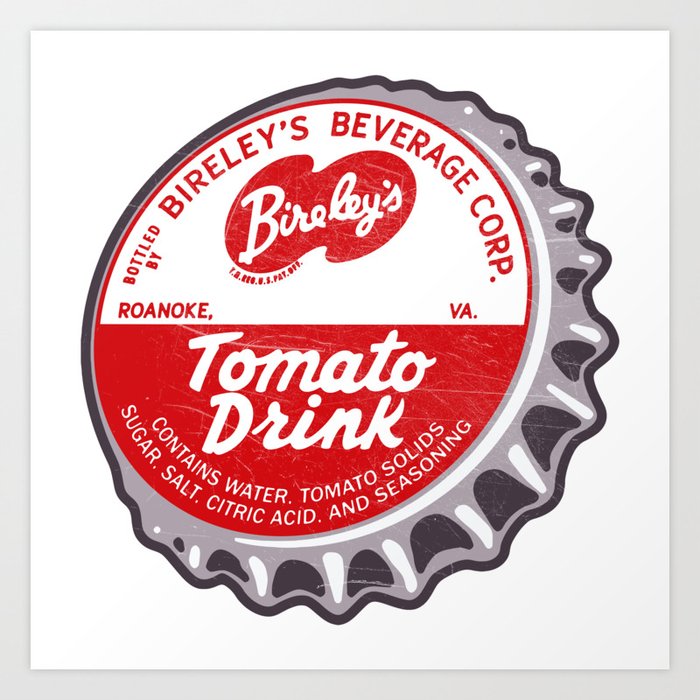This is an illustration of a vintage-style silver bottle cap, showcasing detailed artistic shading with dark gray lowlights and pure white highlights around its scalloped edges. The cap is presented against a white background, occupying the majority of the centered framed image with a light gray border. The cap features a bold, classic design reminiscent of the 1950s or 1960s artwork, divided into two distinct halves. The upper half of the cap has a white background with "Briley's Beverage Corp." in prominent red text along with the Briley's logo at the center, and "Roanoke, VA" on either side of the logo. The lower half is a vibrant red, displaying "Tomato Drink" in large white text, followed by a detailed list in smaller white text along the edge: "Contains water, tomato solids, sugar, salt, citric acid, and seasoning." The entire piece is stylized as a cartoon, adding a nostalgic charm to the presentation.